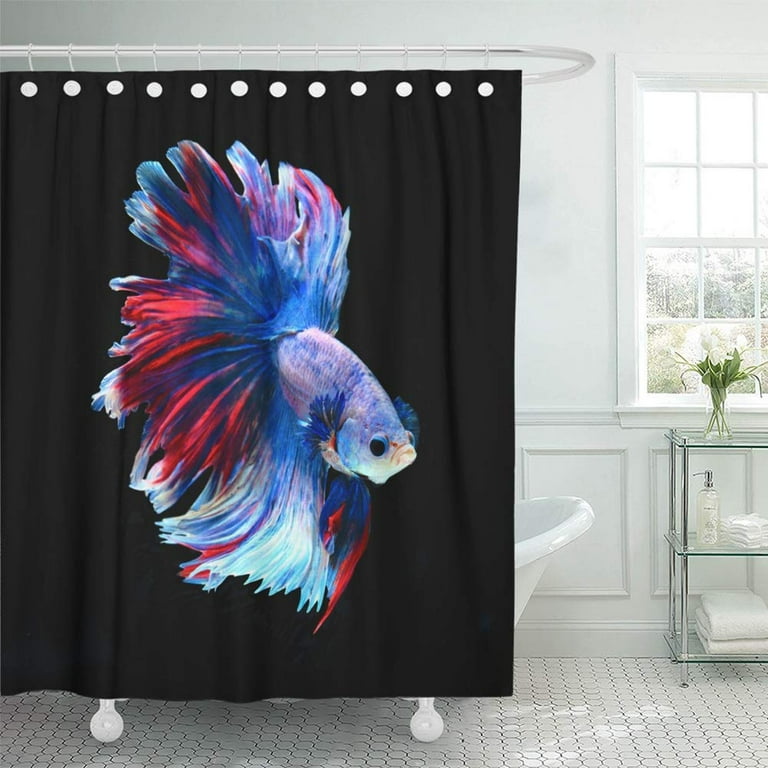This detailed photograph depicts a bright, white-tiled bathroom featuring a prominent white clawfoot bathtub. Centered above the tub is a striking black shower curtain adorned with a vivid Siamese fighting fish design. The fish is depicted in a mix of deep purples, rich reds, various shades of blue, and touches of yellow, with fins that fan out like feathers or ribbons, creating a stunning centerpiece against the black backdrop. The shower curtain is hung on a circular silver rod with hooks that have white clips.

To the right of the tub stands a sleek chrome storage unit with three glass shelves. The top shelf displays a glass vase with a bouquet of white flowers, possibly lilies or roses. The middle shelf holds a pump bottle and neatly tied washcloths, while the bottom shelf contains folded white towels. Above the storage unit is a window that allows natural light to flood the space, casting a warm glow over the predominantly white decor. The bathroom exudes a clean and airy feel, contrasting sharply with the bold, colorful fish design on the shower curtain.